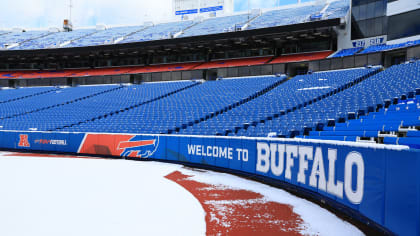The photograph captures an up-close view of the Buffalo Bills football stadium, with a focus on a snowy field corner and adjacent seating. The field is blanketed in snow, except for some reddish markings near the field’s edge, possibly a running track. The stadium seating is predominantly blue, arranged in two levels, including box seats and regular seating, all of which are empty. Blue pads line the wall separating the field from the stands, adorned with banners that prominently display "Welcome to Buffalo" and the iconic Buffalo Bills helmet logo. Additional banners in red and blue run beneath the second row of seats, contributing to the stadium’s vibrant color scheme. This detailed view highlights a quiet moment in the stadium, with no game in play, encapsulating the stillness of a winter day in Buffalo.